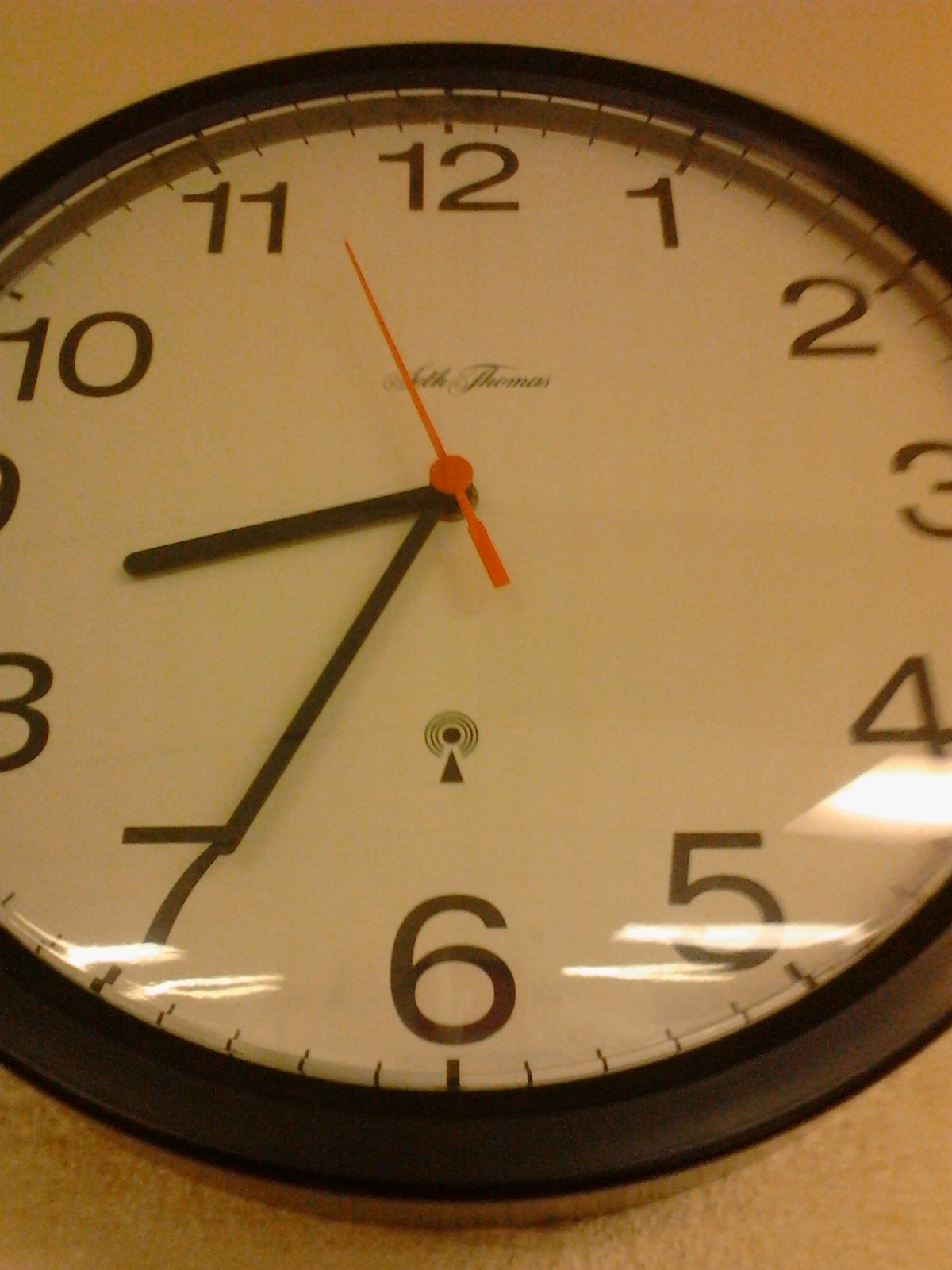This is a close-up photograph of a round analog clock hanging on a wall with a yellow or very light-colored background. Taken from below at a slight angle, the image centers on the clock's face, revealing its distinctive features. The clock has a black frame encasing a typical white face with black numerals, though not all numbers are fully visible—the number 9 is cut from view and only a portion of the number 3 is present. The clock hands are a key detail: the hour hand is positioned between the numbers 8 and 9, while the minute hand points near the 7. Additionally, the red second hand is at about the 57-second mark, pointing between the numbers 11 and 12. The clock face also includes markings for every minute, and faint cursive writing, though the exact words are indiscernible. Notably, the clock is made by Seth Thomas, a detail visible in the cursive writing. The second hand's unique red color contrasts with the black hour and minute hands, adding a striking visual detail.